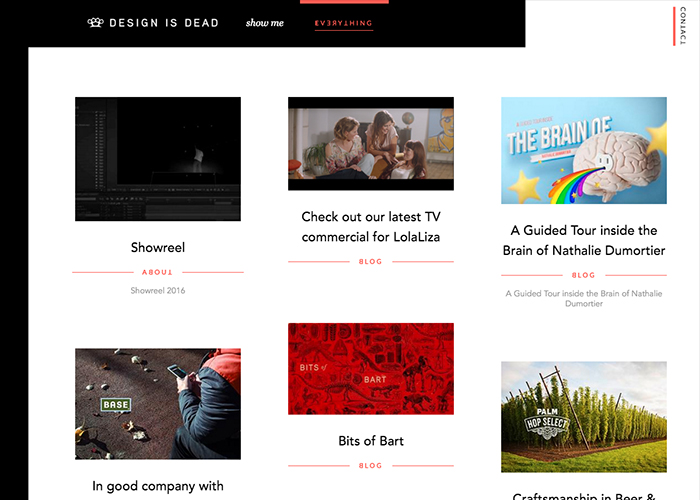Screenshot of a blog website featuring a series of articles with red banners below their titles. The page showcases various articles, each labeled with "Blog" except for the top-left header marked "About." The article titles are in bold black text. The first title on the top left is "Showreel," followed by an article to its right named "Check out our latest TV commercial for Lola Lisa." The next one on the top right is titled "A Guided Tour Inside the Brain of Natalie De Morbery." Below, there are three more articles, but only the middle one is fully visible with the title "Bites Bits of Bark." Each red banner below the titles contains additional text: beneath "Showreel," it reads "Showreel 2016," and under "A Guided Tour Inside the Brain of Natalie De Morbery," it repeats the title.